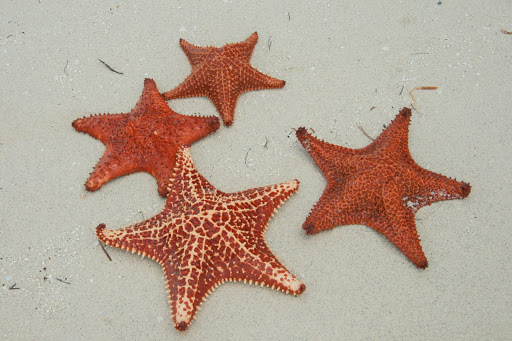This image features a sandy background, potentially a beachfront, with a light gray or white hue interspersed with small pebbles and strands of black and orange debris. Coveted within this setting are four prominently displayed reddish-brown starfish. The most detailed starfish sits prominently at the bottom center of the image, showcasing intricate white lines and fine detailing against its rust-brown surface. To the upper left of this central starfish is a simpler, solid rust-brown starfish, leading upwards towards the top left corner. Adjacent to it on the right is a slightly smaller starfish of a similar solid rust-brown color. In the bottom right corner of the image lies another starfish, notable for its dipped brown tips and subtle white markings on the side of its top right point. The overall composition places emphasis on the detailed textures and varied hues of the starfish against a natural, lightly textured sandy backdrop.